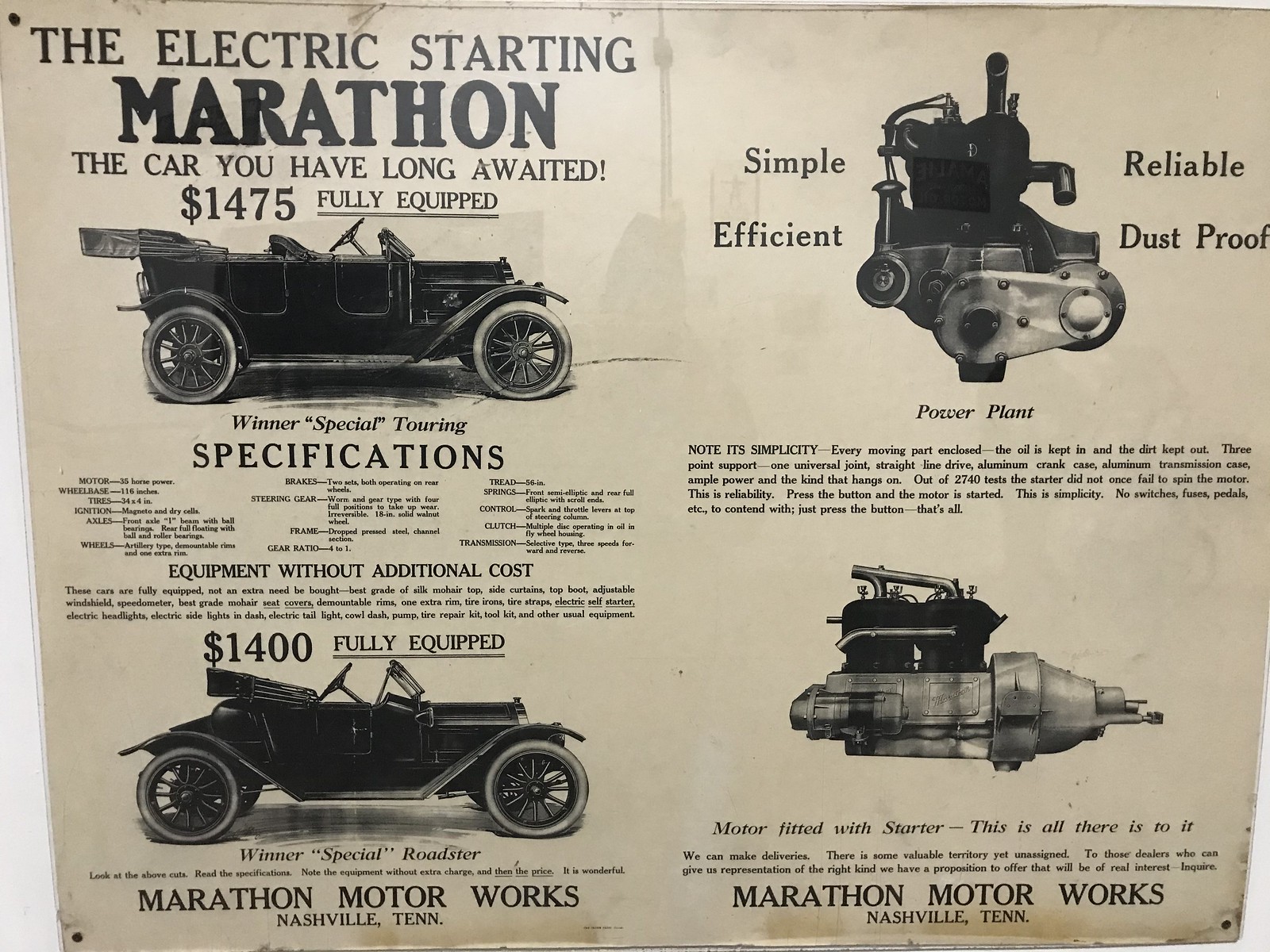This vintage advertisement, mounted against a white wall, features a promotional piece for Marathon Motor Works from the 1920s. The ad, printed on a light brown, parchment-like or faded newsprint material, is divided into four quadrants. In the top left quadrant, bold text announces, "The Electric Starting Marathon – The Car You Have Long Awaited." Beneath this, it highlights the pricing: "$1,475 fully equipped," and touts the vehicle as "simple, reliable, efficient, and dustproof."

The bottom left quadrant displays two images of the automobiles: a special touring version at the top, and a coupe roadster at the bottom. Both versions emphasize that they come fully equipped without additional cost. The text further elaborates on reliability, noting that out of 2,740 tests, the starter never failed to spin the motor. 

On the right-hand side, the top quadrant showcases the engine, lauded for its simplicity and efficient design with every moving part enclosed for dustproof operation. The detailed specification includes a three-point support, one universal joint, a straight-line drive, an aluminum crank case, and an aluminum transmission case. The bottom right quadrant exhibits the starter and additional promotional text that underscores its simplicity: "Press the button and the motor is started. No switches, fuses, pedals, etc. to contend with."

At the bottom right, the ad identifies "Marathon Motor Works, Nashville, Tennessee," reinforcing the brand and its location.